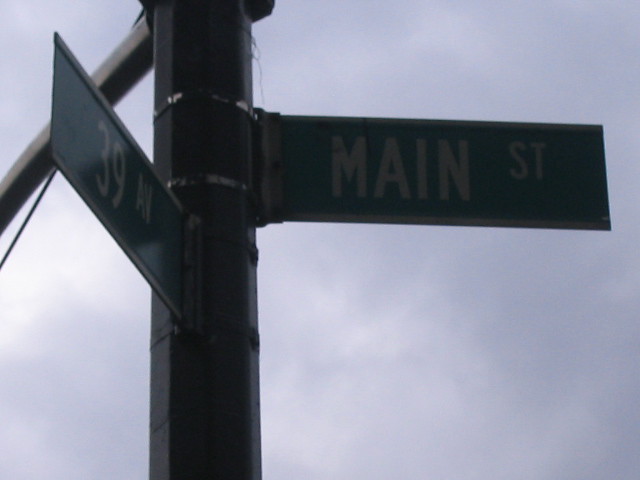In this image, a black street sign pole occupies the left side of the frame, rising to support two individual street signs positioned at its top, extending in opposite directions. The sign facing left clearly reads "Main Street" with white lettering set against a green background. Opposite it, the other sign reads "39 Avenue," also in white letters on a matching green background. The entire scene is set outdoors, under a clouded sky which serves as the backdrop, emphasizing the elevated position of the street sign. No other signage is present in this composition, highlighting the intersection of Main Street and 39 Avenue as the focal point.